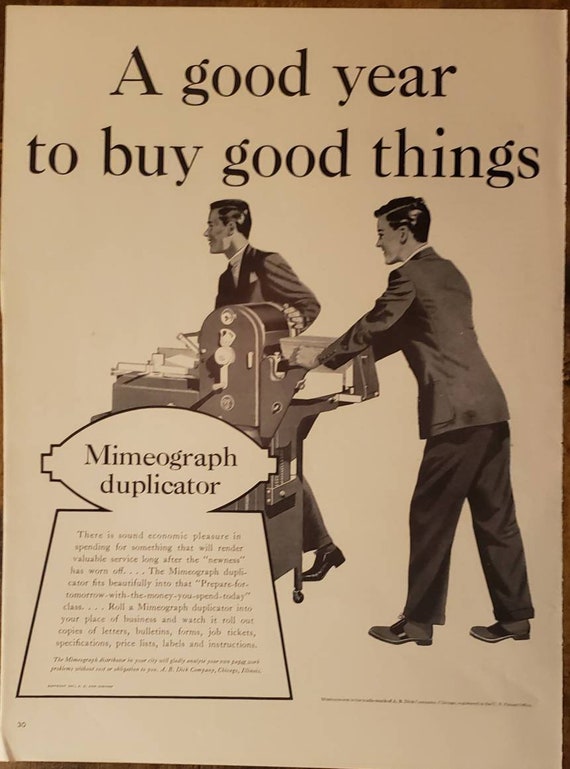The black-and-white, sepia-toned photograph appears to be from an older magazine or advertisement and features a stylized drawing. At the top of the page, bold black text reads, "A Good Year to Buy Good Things." Centrally, the image shows two men, both smiling and dressed in blazers paired with turtlenecks. They sport slick, side-parted black hair and are pushing a gray metal machine—a mimeograph duplicator. One man pushes from the back while the other assists from the side. A distinctive, football-shaped speech bubble prominently displays the words "Mimeograph Duplicator." Below it, a trapezoidal-shaped textbox contains descriptive paragraphs, explaining that the machine can produce copies of letters, bulletins, forms, job tickets, specifications, price lists, labels, and instructions. In the lower left-hand corner, a brief description reiterates "mimeograph duplicator," while very small text in the bottom right corner possibly provides citation or additional information about the picture or the machine. The background is plain, focusing entirely on the men and the machine.